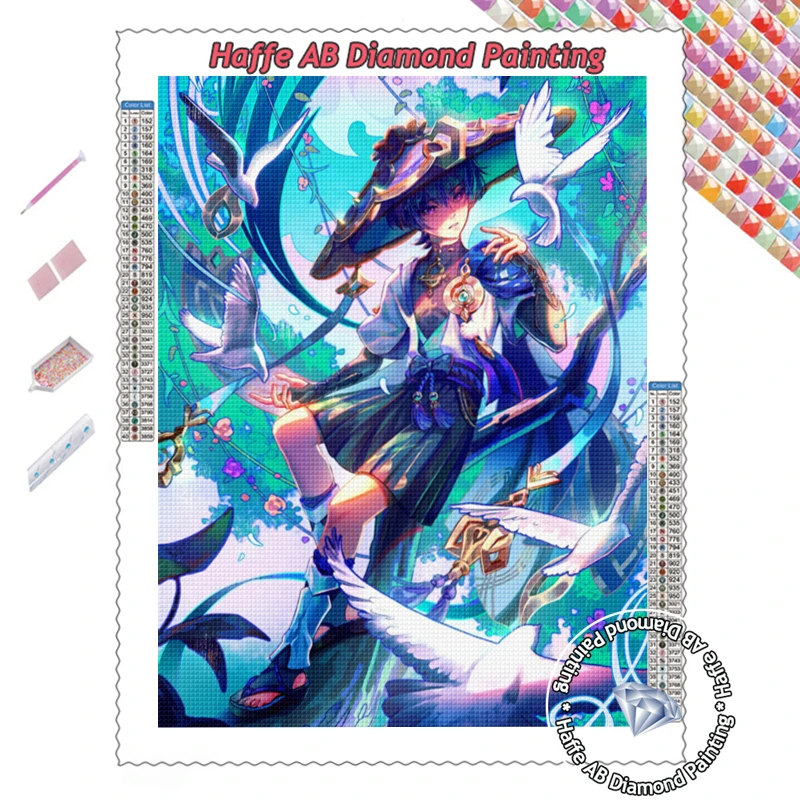This image features a distinctive serrated border reminiscent of a postage stamp. Inside, a white border frames a fantasy-like painting. At both the top and bottom, the text "Haffe A-B Diamond Painting" is displayed in red, with Haffe's name also encircled in the bottom right corner. The scene within this border depicts a whimsical, anime-inspired figure, possibly androgynous, adorned in a wide-brimmed, flowered hat that hints at Thai influences. The figure is dressed in a flowing blue top, a darkish green, Scottish-like skirt, and traditional Japanese sandals. They are poised gracefully on a tree branch, surrounded by an array of white doves, ribbons, and a colorful, multihued background of greens, oranges, purples, and pinks. Glow emanates from both the figure and the birds, adding a magical touch. The overall design, peppered with random beads and numbers, completes the vibrant and dynamic composition.